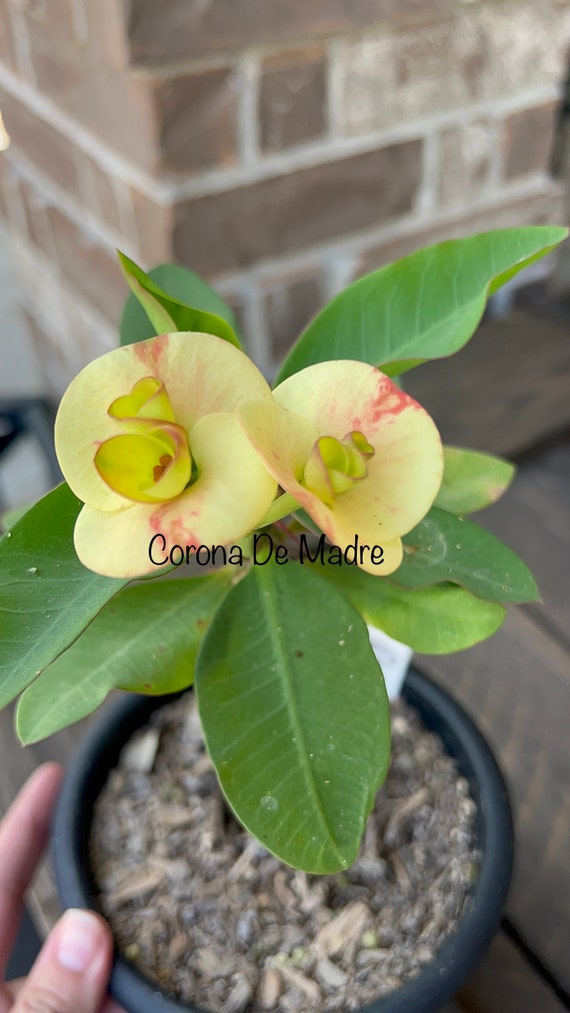This is a detailed close-up photograph of a potted plant situated at the center of the image. The potted plant, held on the left side by a woman's hand with only her thumb and two fingers visible, is in a small black pot filled with mulchy potting soil. The foliage consists of numerous green leaves, and prominently at the top of the plant, there are two small flowers with yellow petals tinged with red, and a distinctive coiled green center. A white tag is visible in the soil. Written in black font across the plant, it says "Corona de Madre." The background features a blurred view of a brick structure, likely a corner of a home, and what appears to be a wooden deck. The perspective of the photo is from above, looking slightly down onto the plant.